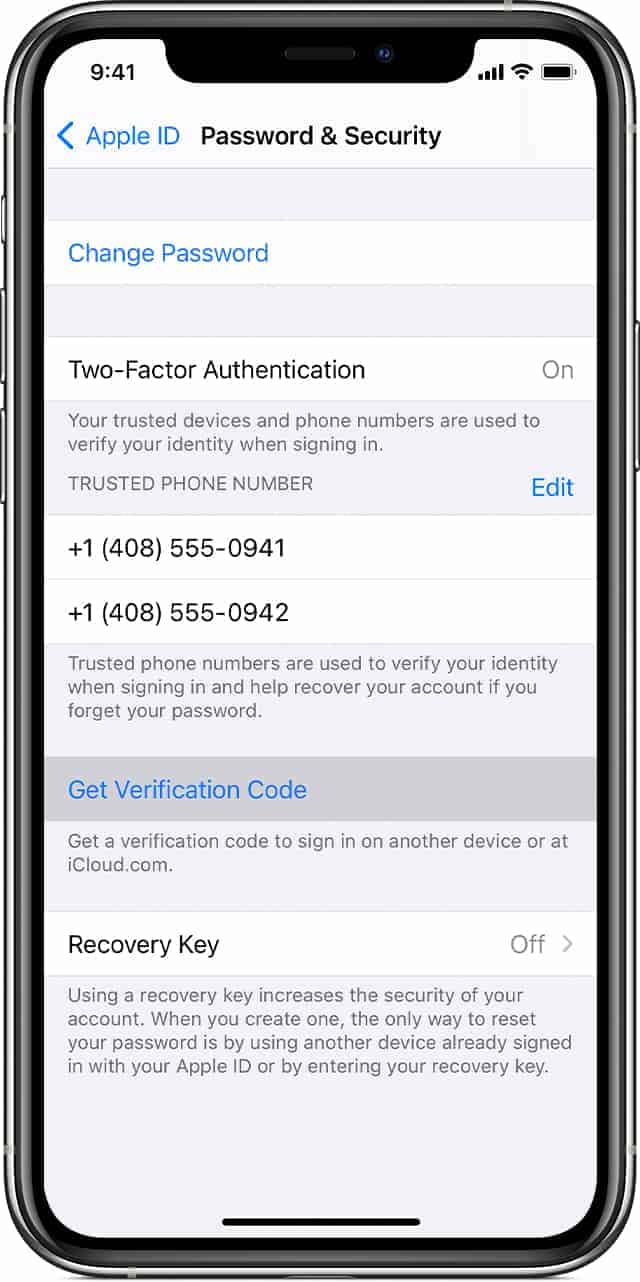The image is a vertically rectangular photograph of a cell phone screen, encased in what appears to be a gray, black, or silver frame. The top of the display shows a white background with status indicators on either side: the time "9:41" on the left, followed by the bar signal, Wi-Fi, and battery icons on the right. The screen content is a section from the Apple ID settings, focused on security features.

The main heading reads "Apple ID", followed by sections for "Password and Security". A link beneath this heading allows the user to change their password. Below, the screen indicates that two-factor authentication (2FA) is enabled, explaining that trusted devices and phone numbers are used to verify the user's identity during sign-in. The detailed section lists two trusted phone numbers, "+1 (408) 555-0941" and "+1 (408) 555-0942", each with an option to edit.

A blue link beneath the phone numbers offers a way to obtain a verification code for signing in on another device or via iCloud.com. The last section on the screen is about the recovery key, noting that this feature is currently turned off. The detailed explanation states that using a recovery key can enhance account security, and it highlights the conditions under which a recovery key can be used to reset the password.